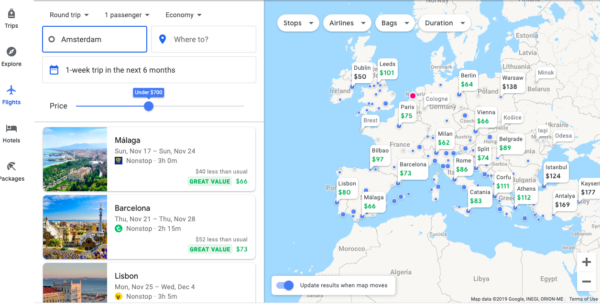**Screenshot Description: Travel Planning Interface**

On the right side of the screenshot, there is a detailed map of Europe with several blue dots representing different cities. Some of these blue dots have speech bubbles extending from them, displaying the name of the city in black text along with a corresponding flight price in green. Not all blue dots have these speech bubbles; only a select few do.

The left side of the screenshot features a vertical panel at the top, which indicates travel details: "Round Trip," "One Passenger," and "Economy." Below that, the travel itinerary states the origin as "Amsterdam," with the trip duration specified as one week within the next six months, and the budget capped at under $790.

The panel presents three highlighted travel options:
1. **Magaluf**: From Sunday, November 17th to Sunday, November 24th. This nonstop flight has a duration of three hours and is priced at approximately $66. It is marked with a "Great Value" tag.
2. **Barcelona**: From Thursday, November 21st to Thursday, November 28th. The nonstop flight lasts two hours and fifteen minutes, costing $73. This flight also carries the "Great Value" distinction.
3. **Lisbon**: From Monday, November 25th to Wednesday, December 4th. This option offers a nonstop flight with a duration of three hours and five minutes, priced at $78.

Additionally, an icon column is located to the left, featuring buttons for "Trips," "Explore," "Flights," "Hotel," and "Packages," with "Flights" highlighted in blue. The destination origin, "Amsterdam," is also boxed in blue.